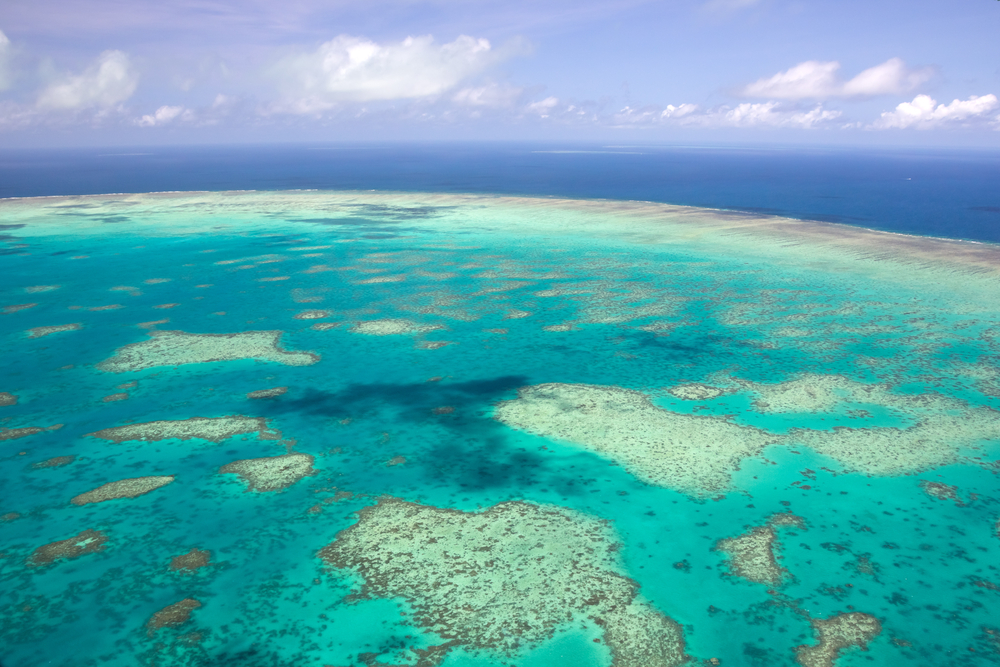This stunning aerial photograph captures a vast ocean scene, likely taken from an airplane. The image beautifully contrasts different shades of blue, with the lighter hues dominating the front two-thirds of the frame and gradually transitioning to darker shades towards the horizon. The lighter blue sections are flecked with patches of sea foam, resembling continental shapes from a bird's eye view. This intricate pattern extends from the foreground towards a darker expanse of ocean, where a distinct, white, foamy line indicates a break point, potentially a wave or tidal movement.

Higher up in the composition, you can see the expansive ocean proper, which appears to continue beyond an arcing reef visible just below the surface. The reef, running from left to right and occupying about three-quarters of the image, shows no signs of human presence—no ships, structures, or people are observable. The colorful waters of the reef, teeming with various shades of green and teal, give way to the deep, uninterrupted blue ocean.

In the background, a clear blue sky dotted with white clouds completes this serene and picturesque scene. The entire composition offers a breathtaking view of nature's beauty, unmarred by human activity, showcasing the stunning interplay of color and texture in the world's oceans.